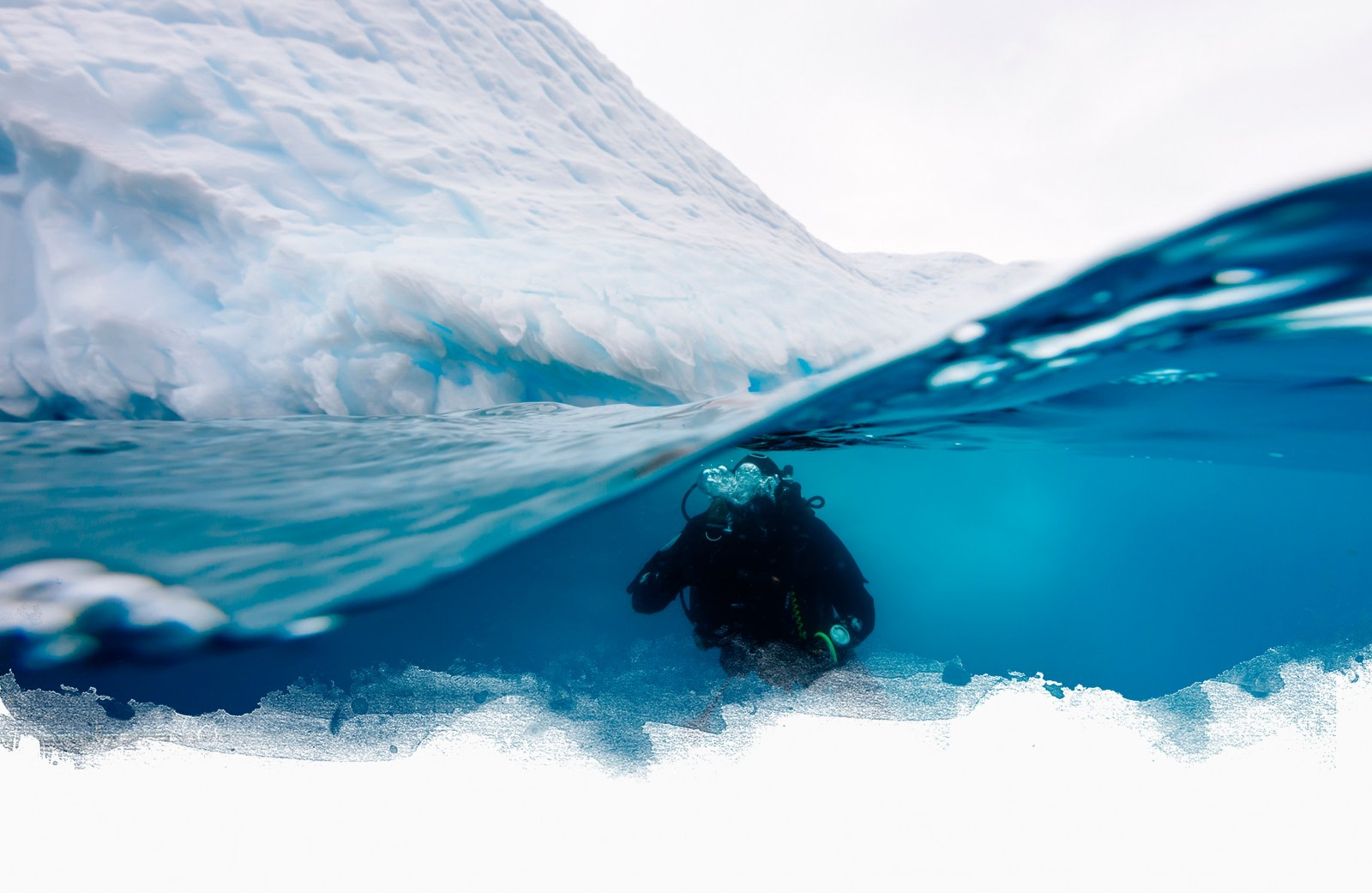This image captures a diver in a black thermal wetsuit, snorkeling beneath a vivid blue, icy water surface. The photograph, skillfully designed to resemble a painting with added artistic paint streaks, presents a striking visual effect. The scene is a cross-section, with the lower part showing the diver underwater and the upper part revealing a clear, white sky devoid of clouds. The diver's face is obscured by bubbles from their respirator, enhancing the feeling of motion and immersion. To the upper left, a massive white wave, possibly edited in with Photoshop, cascades down from the icy shelf or glacier that frames the scene. The icy environment, punctuated by an outcropping of ice, suggests a cold, Arctic setting. The serene blue water below contrasts with the stark, almost surreal white and blue hues of the ice above, creating a compelling and atmospheric composition.